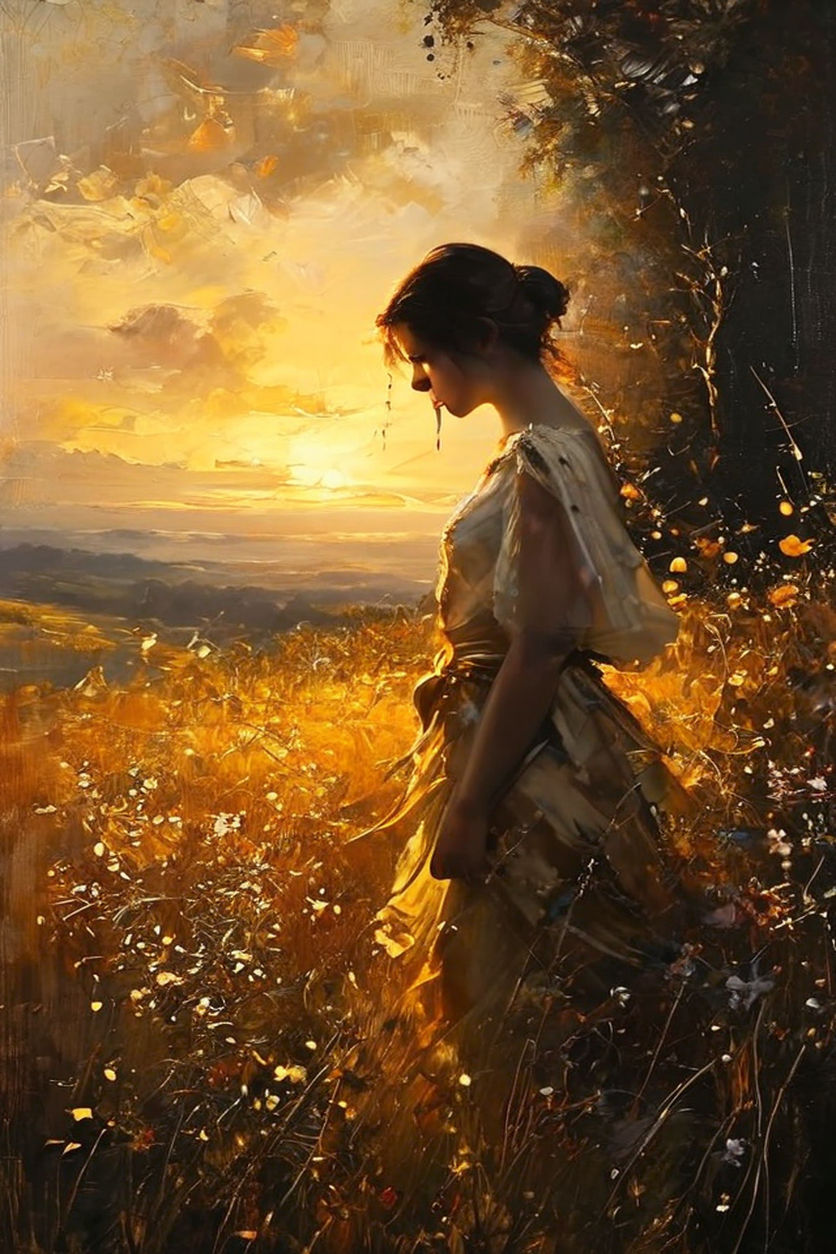In the painting, a young woman stands in a field of tall, golden plants, bathed in the warm glow of a setting sun. Her profile is captured from the left, revealing her contemplative downward gaze. She wears a long, white dress with a printed front, and her brunette hair is styled in a sort of bun. Her left hand rests by her side as she meanders through the golden field, surrounded by rich hues of gold that dominate the scene. In the background, a distant mountain and a valley emerge under a sky tinged with shades of light blue and the deeper tones of a setting sun. Above her right shoulder stands a tree and a bush, adding darker, earthy contrasts to the luminous landscape. The scene is further accentuated by clouds gathering near the horizon and sparkling highlights on various flowers and leaves, adding a touch of fantasy to this serene and evocative illustration.